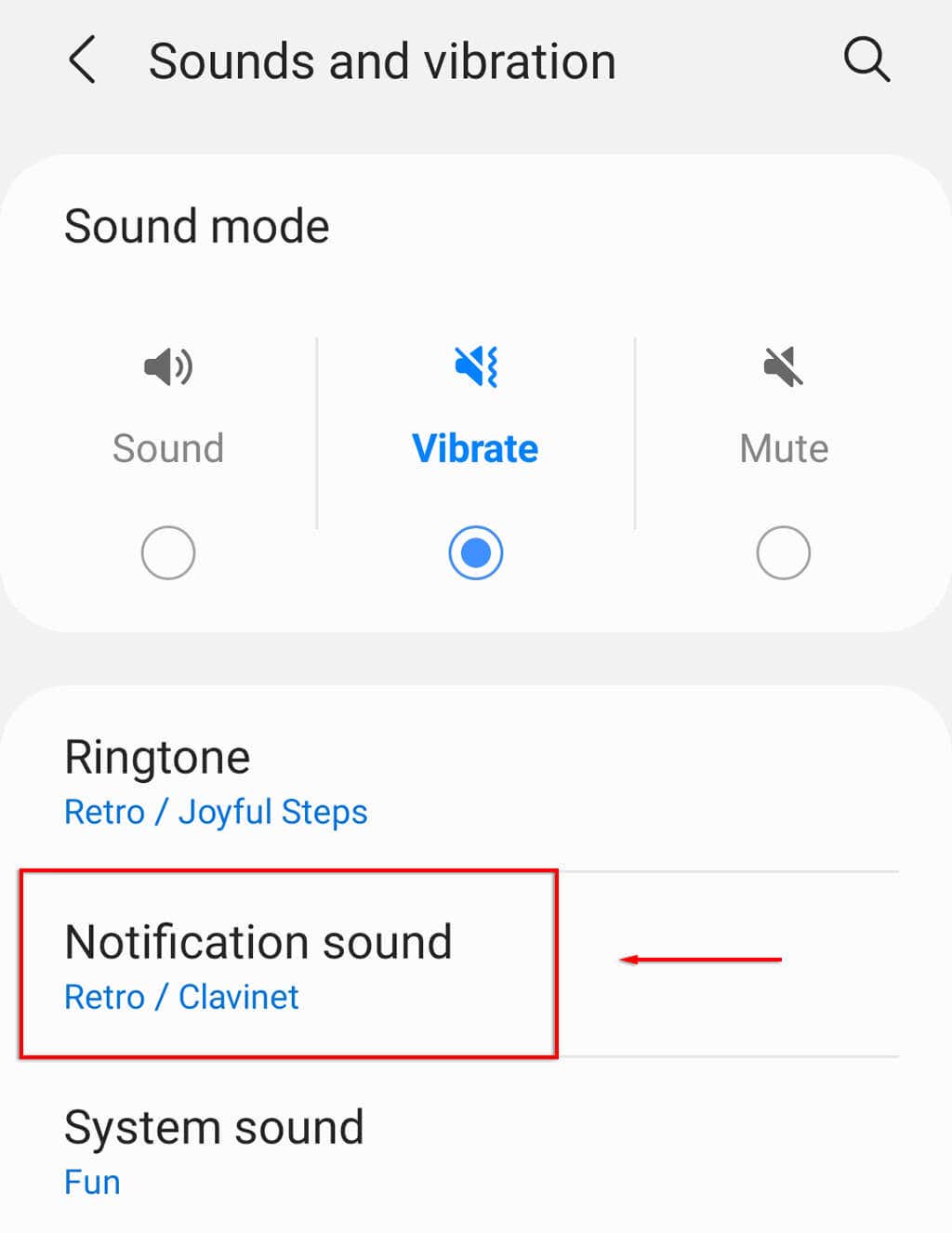The image showcases a mobile phone screen focused on sound settings. 

At the top of the screen, against a light gray background, there is an arrow pointing left accompanied by the text "Sounds and Vibrations." In the top right corner, there is a magnifying glass icon indicating a search function.

Just below, on a lighter gray background, the heading "Sound mode" is displayed. On the far left, there is an icon of a speaker emitting sound waves. Below this icon, the word "Sound" is written, and beneath that is an unmarked circle.

Next to this, a blue microphone icon with a diagonal line through it represents the "Vibrate" mode, indicated in blue text below the icon. Underneath this icon is a circle with a blue center.

On the far right of this line is a gray microphone icon, also with a diagonal line through it, representing the "Mute" mode. The word "Mute" is written beneath this icon, with an unmarked circle underneath.

Further down, the screen displays "Ringtone" in black text. Underneath, in blue text, the selected ringtone is named "Retro/Joyful Steps."

Below the ringtone information, there is a black text label "Notification sound." Beneath this label, blue text reads "Retro/Clavinet," surrounded by a red border. A red arrow points directly at this text, highlighting it.

Finally, the "System sound" setting is indicated in black text, with the word "Fun" written in blue directly beneath it.